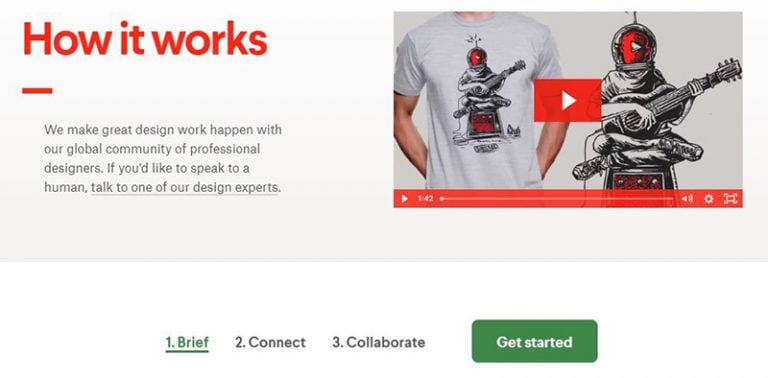A screenshot of a web interface detailing a design service workflow. On the left side, the title "How it works" is prominently displayed in red text. Below it, a dashed line extends under the letter 'H' and then leads into a descriptive section that reads, "We make great design work happen with our global community of professional designers. If you'd like to speak to a human, talk to one of our design experts," with the phrase "talk to one of our design experts" underlined for emphasis.

Adjacent to this text, on the right, is an embedded YouTube video. The video features a man in a t-shirt which depicts a person wearing a red helmet, playing a guitar, seated cross-legged on a speaker. The red play button is visible in the center of the video, with a red play bar at the bottom.

Next to the video, a larger version of the t-shirt's graphic is displayed, emphasizing the artistic design. Beneath these visuals are four options laid out horizontally: "Brief," "Connect," and "Collaborate." The word "Brief" is highlighted in green text and underlined, indicating its selected status, while the other options are presented in gray.

On the far right, there's a green rectangular button with white text that reads "Get Started." The background of the interface is predominantly white, and there are no visible headers, branding, logos, or company names, suggesting this might be a prototype or a screenshot from a browser interface. It remains unclear if this was captured from a live website or is simply a mock-up design.